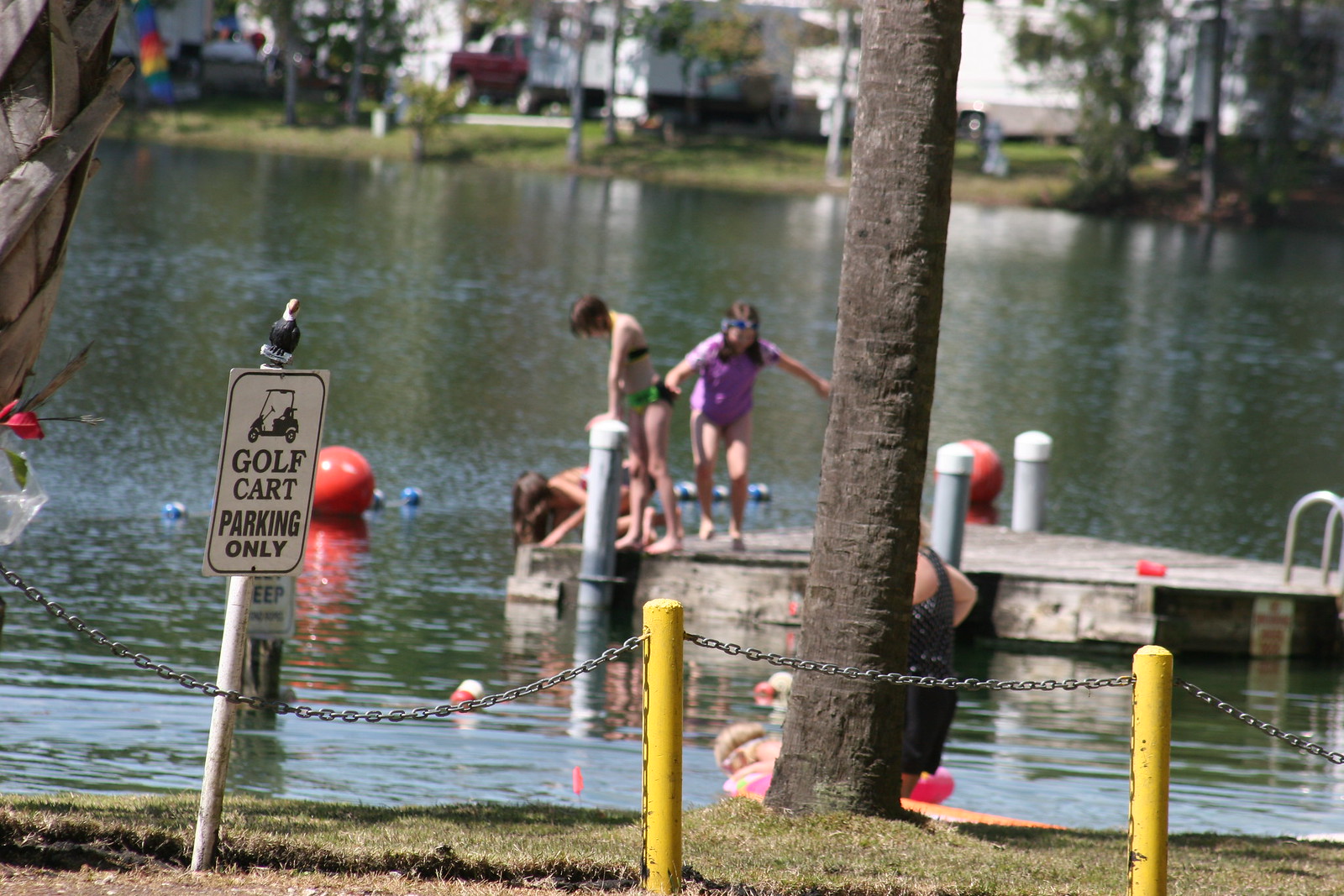In this full-color photograph taken outdoors during daylight, likely in summer, the scene captures a lively lakeside campground setting. Prominent in the image are three children playing on a wooden pier or dock, with two standing near the end and one crouching at the very tip, all positioned toward the middle distance. Framing the foreground, there are several yellow posts connected by chains, enclosing a grassy area. A black and white sign reads "golf cart parking only," and a black and white bird perches atop it, adding a touch of nature to the scene. 

Off to the left, partially visible, is the back of a woman standing near the beach. The foreground also features a grayish tree trunk extending out of the frame's top. On the far left at the top of the image, a partially obscured wooden object can be identified. Across the lake in the background, the water glistens with greenish-gray hues enriched by blue highlights from the sun. Distantly, some trailers and a red truck can be seen, indicating the presence of other campers, cementing the atmosphere of a bustling summer campground.